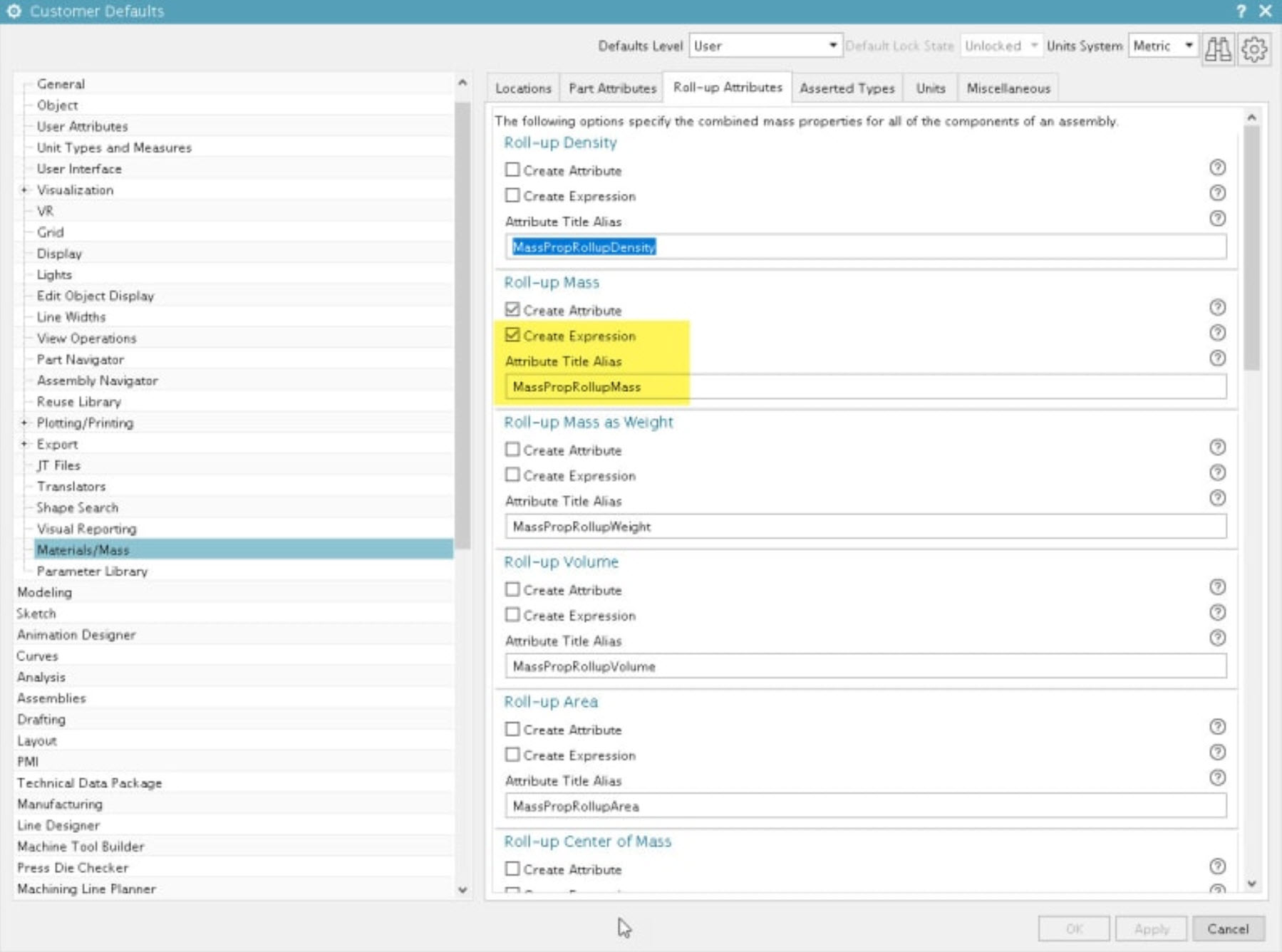This detailed caption describes a complex user interface showcasing various settings and options:

---

The image depicts an extensive menu interface with numerous clickable tabs categorized under different sections, providing options for customizing customer defaults. On the left panel, the categories include: General, Object, User Attributes, Unit Types and Measures, Screen or Interface, Visualization, VR Grid, Display, Lights, Edit, Object Display, Line Widths, View Operations, Part Navigator, Assembly Navigator, Reuse Library, Plotting/Printing, Export, JT Files, Translators, Shape Search, Visual Reporting, Material, Mass Parameter Library. Further down are additional categories: Modeling, Sketch, Animation, Design, Curves, Analysis, Assemblies, Drafting, Layout, PMI, Technical Data Package, Manufacturing, Line Design, Machine Tool Builder, Press Die Checker, and Machine Line Planner.

On the right panel, the top displays options for Default Level, User, and Default Lock State, which is currently set to Unlocked. The Unit Systems is set to Metric. Next to these options are icons of a Binocular and a Gear (Wheel).

Below, the sections include Locations, Part Attributes, Roll Up Attributes, Asserted Types, Units, and Miscellaneous. The text indicates that the following options specify and combine the mass properties for all components of an assembly: Roll Up Density, Create Attribute, and Create Expression. There are two achievable checkboxes here, marked with question marks next to them.

Further sections include titles like Attribute Title On The Out, Alias, Mass, Probe, and Roll Up Density, with subsequent options such as Roll Up Mass. This section lists options like Create Attribute and Create Expression, both checked, alongside titles marked in yellow. Roll Up Mass displays as Weight, with the same checked options and titles reiterated.

Proceeding, there is a Roll Up Volume section with unchecked boxes for Create Attribute and Create Expression, and similar layouts with attributes such as Alias, Mass, and Probe. The last sections include Roll Up Area and Roll Up Center Mass, with Create Attribute again unchecked and all accompanied by their respective question marks.

---

This comprehensive description thoroughly outlines the layout and the various functionalities available in the depicted menu interface.